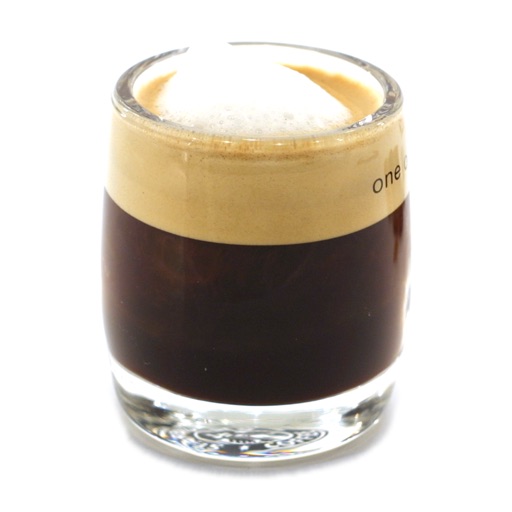The image showcases a small, barrel-shaped glass filled with a richly layered espresso-based drink. The glass, resembling a shot glass but slightly wider and without a handle, contains a dark brown liquid occupying the lower two-thirds of the glass. Above this sits a substantial layer of light brown foam topped with a striking dollop of white foam, slightly cresting over the rim. The glass features the word "one" etched in lowercase black letters on the right side, perfectly clear and easily readable against the otherwise plain, white background. A hint of a shadow beneath the glass adds depth to the image, enhancing the focus on the intricate layering and texture of the drink within the transparent, thick glass material.